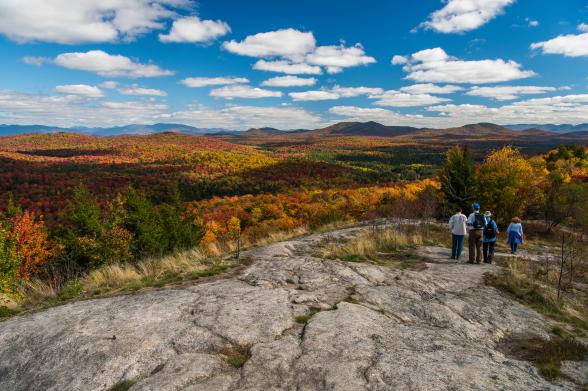The photograph captures a group of four hikers enjoying a scenic outdoor adventure. They are positioned toward the center-right of the image, standing on a grey, rocky surface interspersed with shoots of grass. The diverse trees stretch out for thousands of acres, showcasing a vibrant array of autumn colors, from orange and yellow to red, interspersed with green pine trees.

The hikers, only visible from the back, are dressed in a mix of blue and white outfits. One woman with red hair is wearing a light blue shirt with a blue sweater tied around her waist, while another person in a darker blue shirt also dons a backpack. The remaining two individuals include a person in a white shirt and another in a blue shirt. They are all gazing out at the expansive landscape.

In the background, a distant mountain range adds to the majesty of the scene, under a sky filled with floating, white, fluffy clouds. This picturesque setting underlines the hikers' immersive experience in nature, highlighting their adventurous spirit on this sunny, pleasant day.